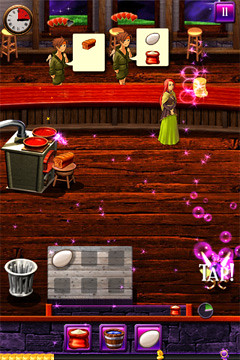The image is a vertical rectangular screenshot from a colorful video game, likely captured on a phone. It depicts the interior of a vibrant and bustling tavern or bar filled with rich red, brownish-red, purple, and lilac hues. The main focus is on two characters standing behind a bar, each with a white box in front of them; one box holds a loaf of bread, and the other contains an egg and flour. Opposite them, a woman with long red hair, dressed in a shawl and a long green skirt, stands by the bar with purple magic bubbles floating around her and a bag of flour on the counter.

In the environment, there is a wooden floor and an oven to the left with a loaf of bread placed on a small wooden stool. The bottom right of the image features a trash can and a rectangular menu displaying six small boxes, with an egg in the first box and the rest empty. Below this menu, the word "tap" appears, accompanied by rising purple bubbles.

The top part of the screen shows three blue windows adorned with red flowers on their sills. The upper-left corner features a small clock with a red segment, indicating time usage, and the upper-right corner has a purple square displaying the number 11. Additional icons at the bottom center of the screen include a purple square for a flour bag, a bowl of water, and a white seed, which are interactive elements of the game. To the middle left, two large pans with red liquid sit on a stovetop. Overall, the scene is digitally illustrated with numerous interactive elements and magical visual effects.